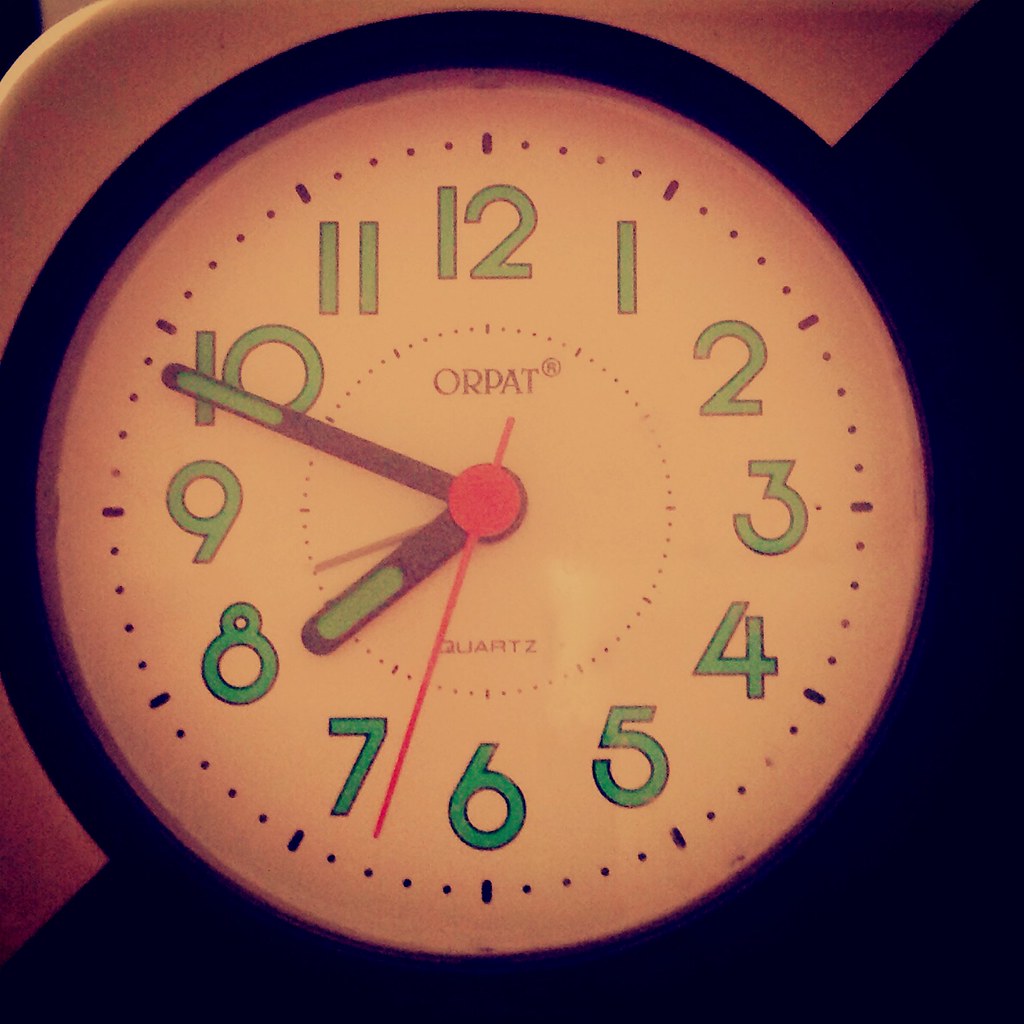This is a highly detailed up-close photograph of a vintage-style wall clock positioned centrally within a square image. The clock features a black border with a white clock face and is set against a backdrop divided diagonally; the top half is reddish-orange, and the bottom half is black. The numbers on the clock are in a bold, block-style font and are teal green in color. The clock's minute and hour hands are predominantly black with a rounded rectangular teal green accent at the ends, while the second hand is red. The face of the clock also includes the brand name "Orpat" at the center, followed by the word "Quartz" beneath it. The time displayed on the clock is 7:49. Each minute mark on the clock is indicated by a dash, appearing every two minutes.